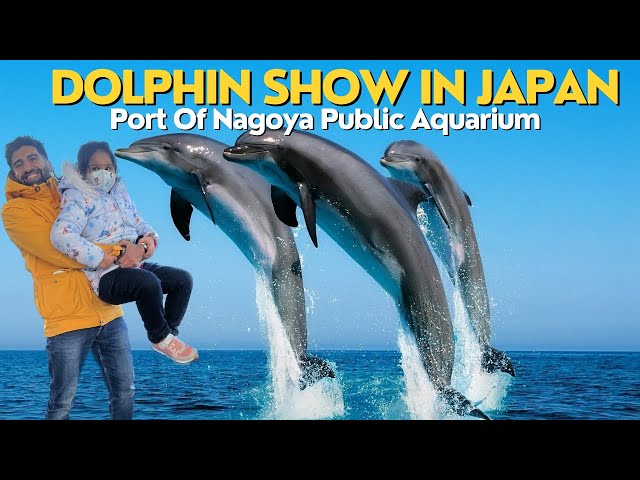The image is an advertisement for a dolphin show held at the Port of Nagoya Public Aquarium in Japan. The ad features vibrant yellow text at the top that reads "Dolphin Show in Japan," with a white subtitle indicating the location of the event. Front and center are three sleek, gray dolphins with white bellies, perfectly synchronized as they leap out of the ocean. The background showcases clear, blue skies, evoking a sense of freedom and excitement. In the left corner, a father in a yellow jacket and blue jeans is holding his young daughter, who is dressed in a multicolored jacket with a light blue background, blue pants, pink shoes, and a face mask. The father smiles warmly, while the daughter's expression is hidden behind the mask. The positioning of the father and daughter appears somewhat photoshopped, suggesting they were added to the corner of the vibrant scene to create a wholesome, family-friendly appeal.